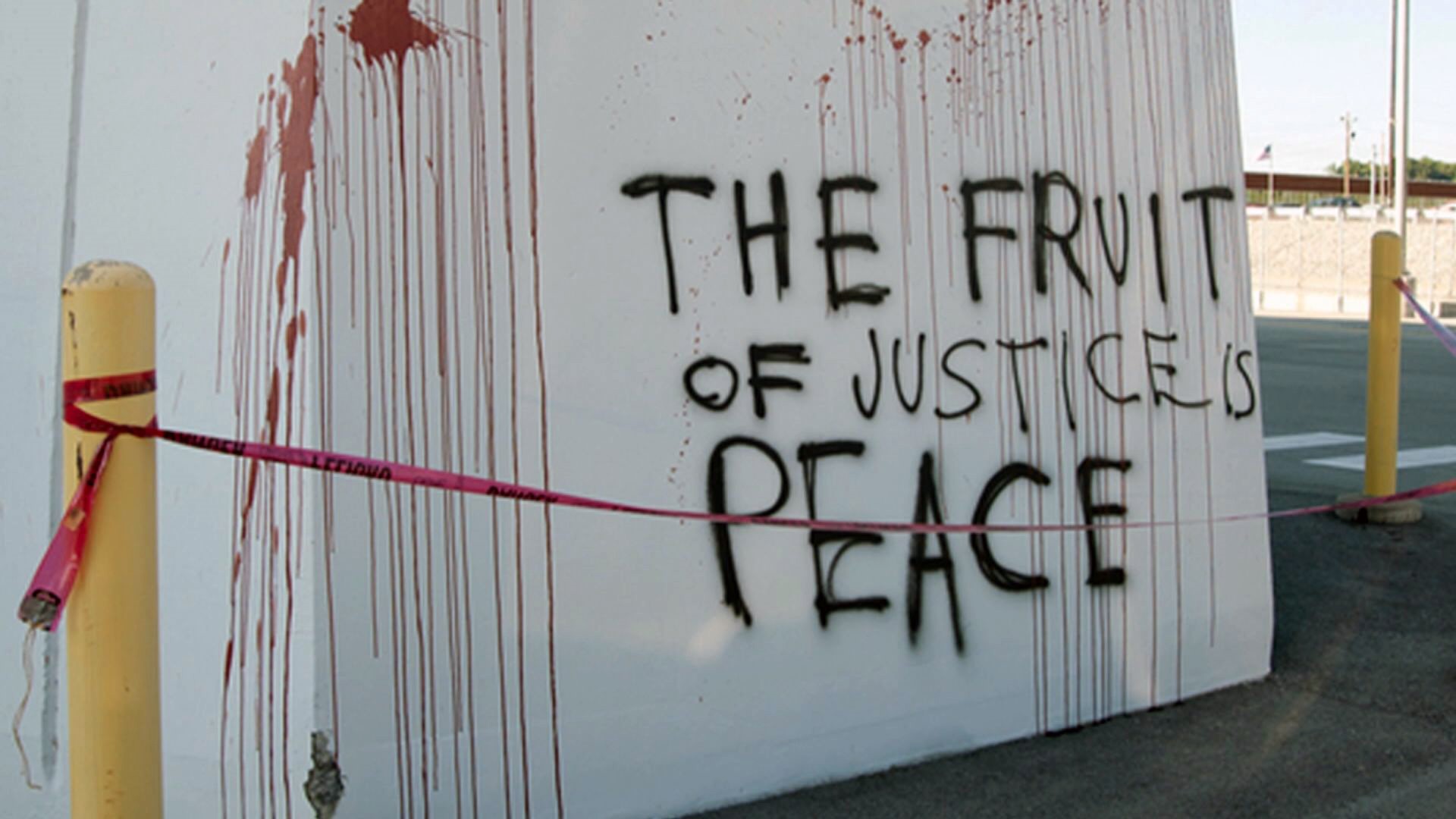This image depicts what appears to be a crime scene or an act of vandalism against a stark white wall. Prominent on the wall are red smears and splatters that look like blood, though they could also be paint or another substance mimicking blood. The words "The fruit of justice is peace" are messily spray-painted in black graffiti across the wall. Two yellow posts anchor a stretch of red crime scene tape that wraps around one post, stretches out of view, and then reconnects to another visible post. The setting seems to be a concrete parking lot, with additional features in the distance, including an American flag and a background that could be a little hill or another parking lot. There's a hint of a crosswalk and possibly a brick wall far off, and some describe a stadium in the background. The overall scene is chaotic and tense, marked by the contrasting bright red against the sterile white wall and marked off by the caution tape.